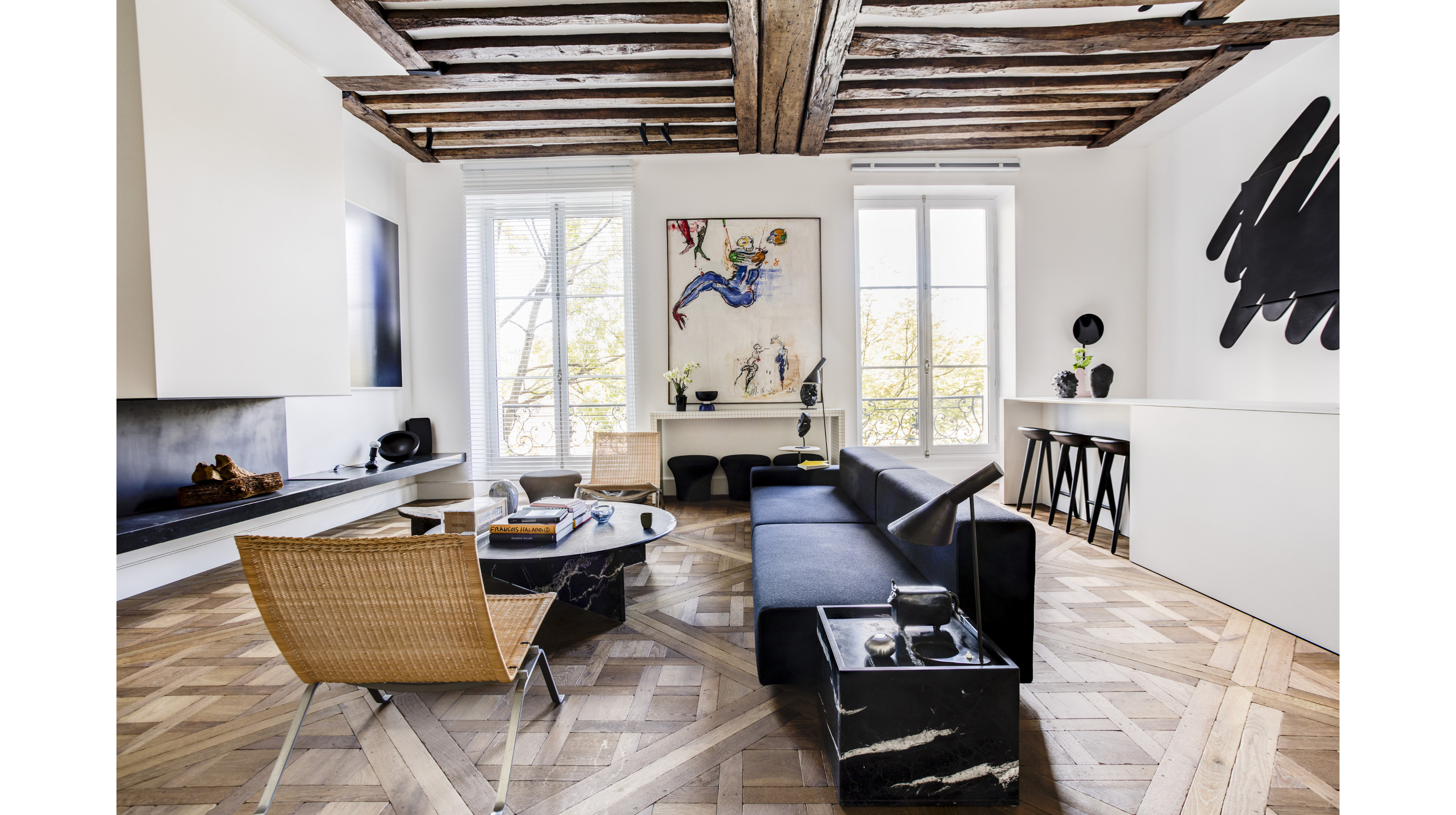The image captures a modern living room with a sleek, black sofa positioned centrally. Flanking this couch is a unique coffee table, combining marble and glass elements atop a black base, adorned with various objects. To the left of the sofa, there's a woven brown wicker chair, offering a cozy seating option. The room's flooring is a distinctive wooden crisscross pattern that adds texture to the space.

The room's gray ceiling features wooden slats running lengthwise, giving a rustic touch amidst the modern decor. The walls are primarily grayish, with expansive windows on either side of the back wall, allowing natural light to illuminate the space. These windows frame a central wall that hosts a large painting above a white table adorned with a flowering plant.

On the opposite side of the sofa, a sleek, modern TV is mounted on the wall, while another wall showcases a contemporary black art piece. The far right wall slightly visible in the image has a distinctive, large black scribble artwork. This living room is exemplified by a harmonious blend of modern and rustic elements, making it both functional and aesthetically pleasing.